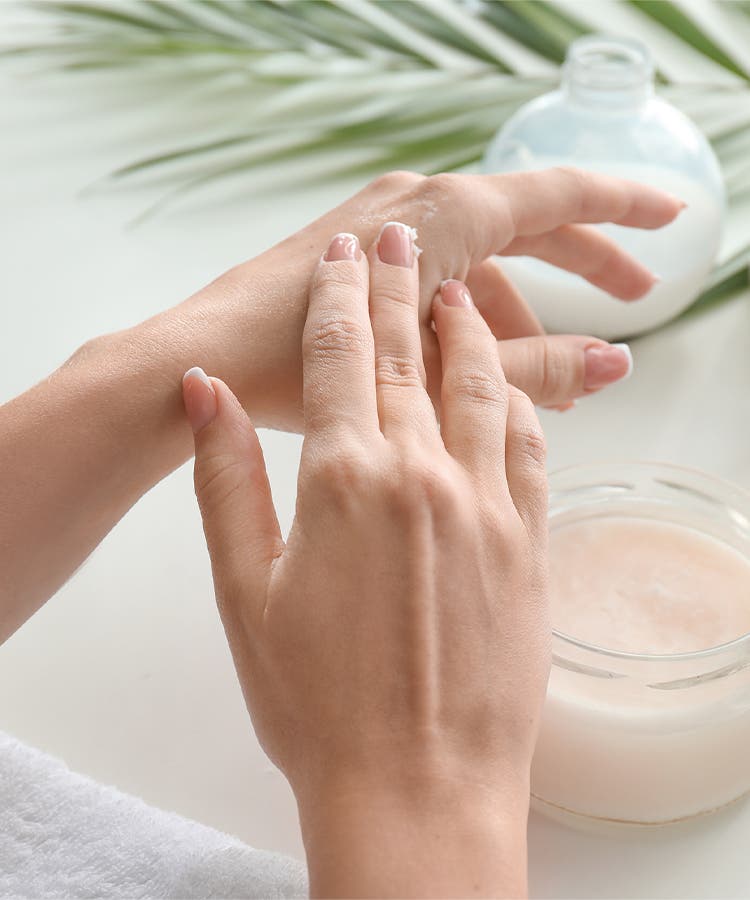The professional color photograph captures a luxurious and serene spa-like atmosphere, featuring a woman with perfectly manicured hands applying a thick body butter cream. Her right hand, emerging from the bottom of the image, displays neatly polished nails with a subtle pink and white French manicure as it delicately spreads the cream on her left hand, which enters gracefully from the left side. Both hands showcase smooth, light-colored skin, free of rings, suggesting a Caucasian or possibly Asian ethnicity.

A clear glass jar containing the thick, slightly pink-tinged cream is prominently positioned in the bottom right corner. In the blurred background, a spherical, globe-like bottle without a lid is visible, adding to the sense of high-end skincare. The setting includes a fluffy white towel in the bottom left corner and elegant green palm fronds spanning the upper part of the image, enhancing the spa ambiance. The overall composition, marked by clean off-white surfaces and a soft-focus background, highlights the meticulous skincare ritual, making it suitable for use in advertisements or catalogs for a spa or skincare brand.